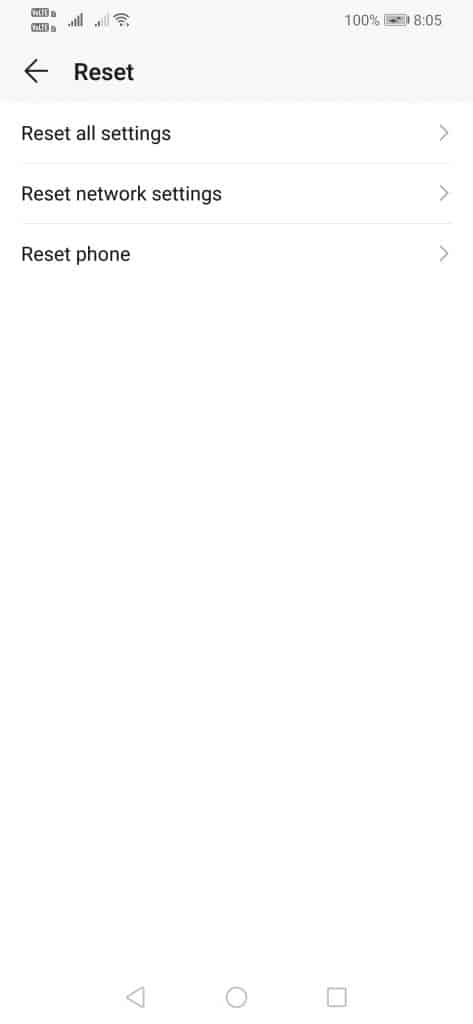A minimalist cell phone screen displaying various settings and status icons. 

- **Top Left Corner:**
  - Two grey status bars stacked vertically, accompanied by a grey lock icon to their right.
  - Four full WiFi signal bars followed by two WiFi signal bars.

- **Top Right Corner:**
  - Signal strength indicator showing 100% in muted grey.
  - Battery icon featuring a lightning bolt, indicating charging.
  - The time displayed as "8:05" on the far right.

- **Mid-Section:**
  - Just below the WiFi icons, a black left arrow and bold text "Reset" pointing to the left with the arrow.

- **Three Main Sections with Headings:**
  - "Reset All Settings" on the left with a right arrow on the far right.
  - "Reset Network Settings" on the left with a right arrow on the far right.
  - "Reset Phone" on the left with a right arrow on the far right.

All headings and arrows are in black on a pristine white background, neatly stacked one atop the other.